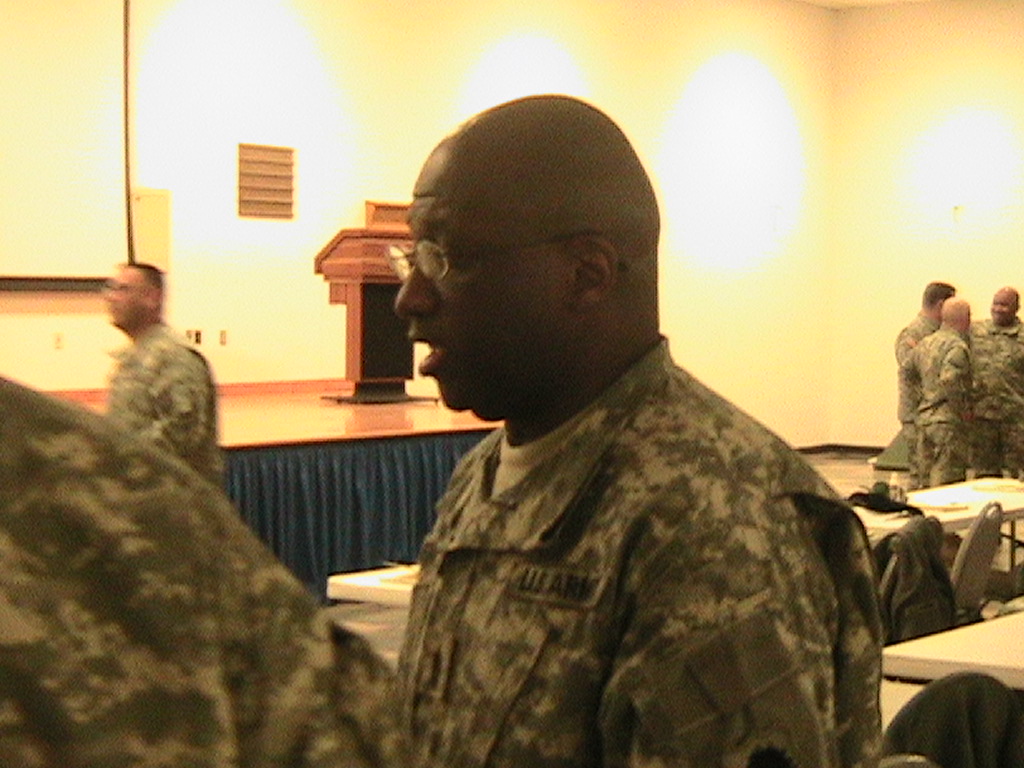This image captures an interior view of a conference room, likely set up for a military event. The room features an elevated stage with a podium, adorned with a blue curtain at the bottom, and a large, unused white projector screen in the upper left-hand corner. In front of the stage, there are two rows of white desks and folding chairs, some of which have coats draped over them and papers or folders scattered on their surfaces. The setting suggests that the event is either about to commence or has just concluded, as there is no one at the podium and the lights are fully illuminated.

In the foreground, a bald African-American man with round glasses stands, wearing a green camouflage army uniform with a bar indicating "U.S. Army" on it. He wears a green t-shirt beneath the camouflage. Alongside him in the foreground, there are three other individuals interacting, all donned in similar head-to-toe camouflage attire. In total, six people in military fatigues are visible in the image, indicating their likely affiliation with the U.S. Army. One individual is seen walking towards the projection screen at the back. Additionally, the wood flooring of the stage displays a visible grain, contributing to the room's detailed setting.